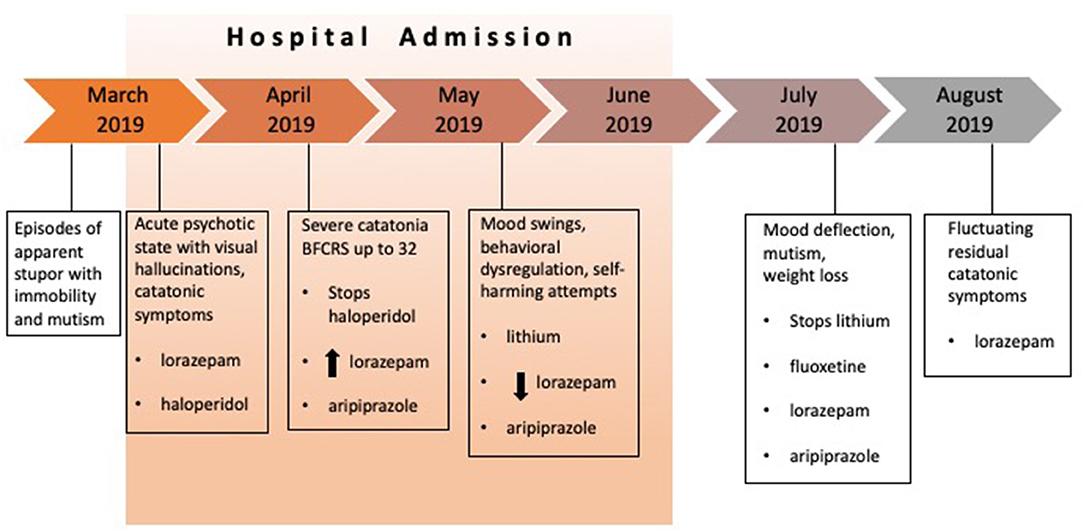The image is a detailed flowchart titled "Hospital Admission," displayed in small black letters. The chart traces hospital admission processes related to behavioral health from March 2019 to August 2019, using arrows to represent the flow of time. The arrows transition in color from orange to gray as the months progress.

At each monthly interval, there are descriptive boxes detailing the patient's condition and treatment. In March 2019, the patient experiences episodes of apparent stupor with immobility and mutism, along with an acute psychotic state marked by visual hallucinations and catatonic symptoms, requiring medications such as lorazepam and hydroxyzine. April sees a severe increase in catatonia, recorded with a BFCRS score of 32, leading to the cessation of hydroxyzine and initiation of adrenal pills.

In May, the patient faces mood swings, behavioral dysregulation, self-harming attempts, and continues on lithium, lorazepam, and acid suppressants. By July, there are mood deflections, mutism, and significant weight loss, prompting a stop to lithium, fluoxetine, and other medications, including lorazepam and aripiprazole. Finally, in August 2019, the patient exhibits fluctuating residual catatonic symptoms and is maintained on lorazepam. Each box not only details the patient's evolving symptoms but also the adjustments to their medication regimen throughout the period.